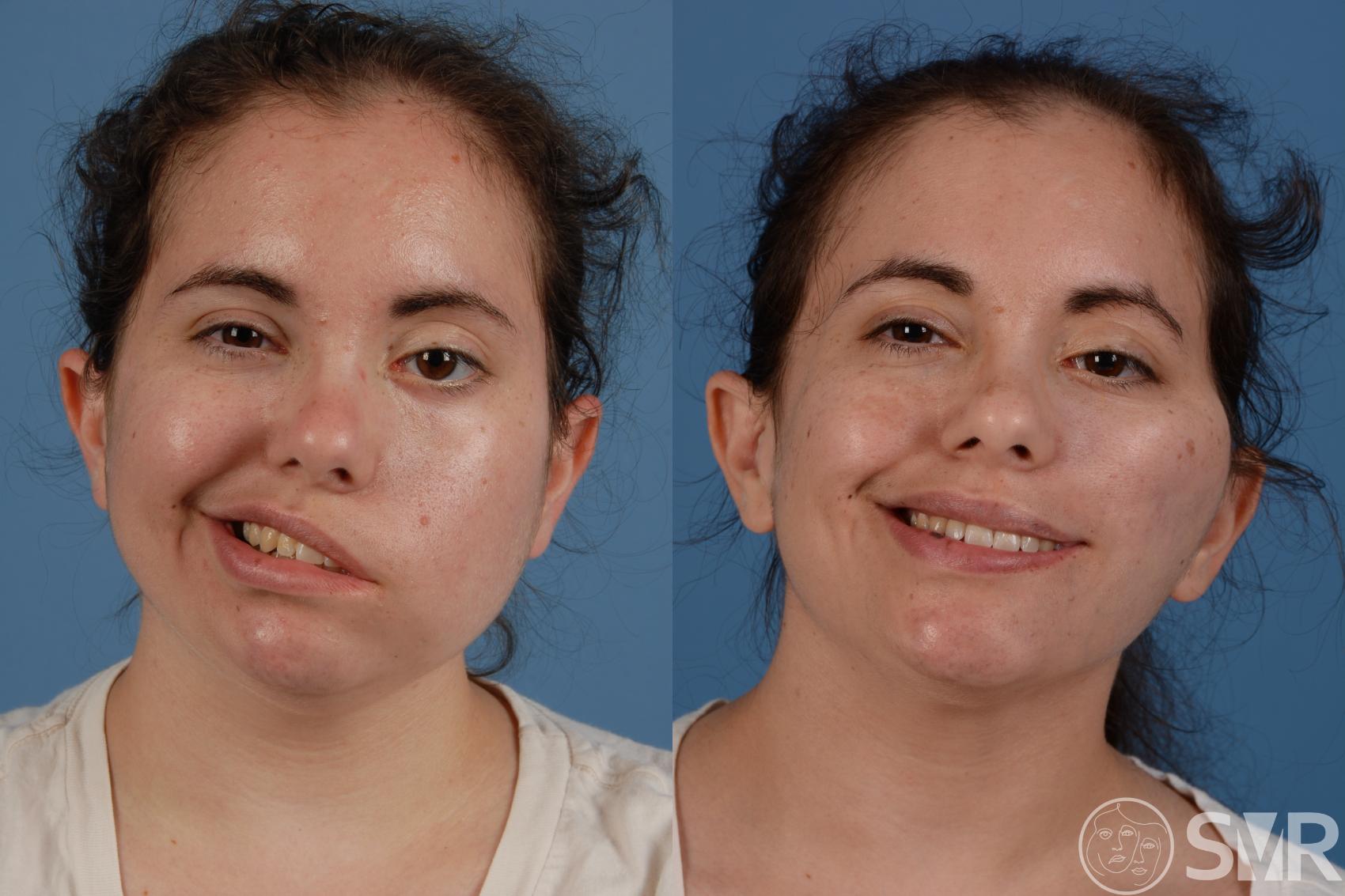The image displays a before-and-after comparison of a young woman in her 20s or 30s with long, curly brown hair pulled back into a ponytail and brown eyes. The photos are set against a light blue background and feature a watermark with the letters "SVR" accompanied by a logo of two faces, suggesting it represents a medical treatment service for facial conditions.

In the 'before' photo on the left, the woman is smiling, but her smile is noticeably asymmetrical. The left side of her mouth is significantly higher than the right, and her left eye appears partially closed, giving her face a pulled and uneven appearance. This may be due to a muscular or neurological condition.

In the 'after' photo on the right, improvements are evident. Her smile is more centered and balanced, with both corners of her mouth lifted symmetrically. Additionally, her left eye is more open, contributing to a more natural, brighter smile. Although there seems to be a slight bump on the left side of her face, potentially due to postoperative swelling, the overall correction is clear. She is dressed in a white shirt in both photos, indicating they were taken relatively close in time.